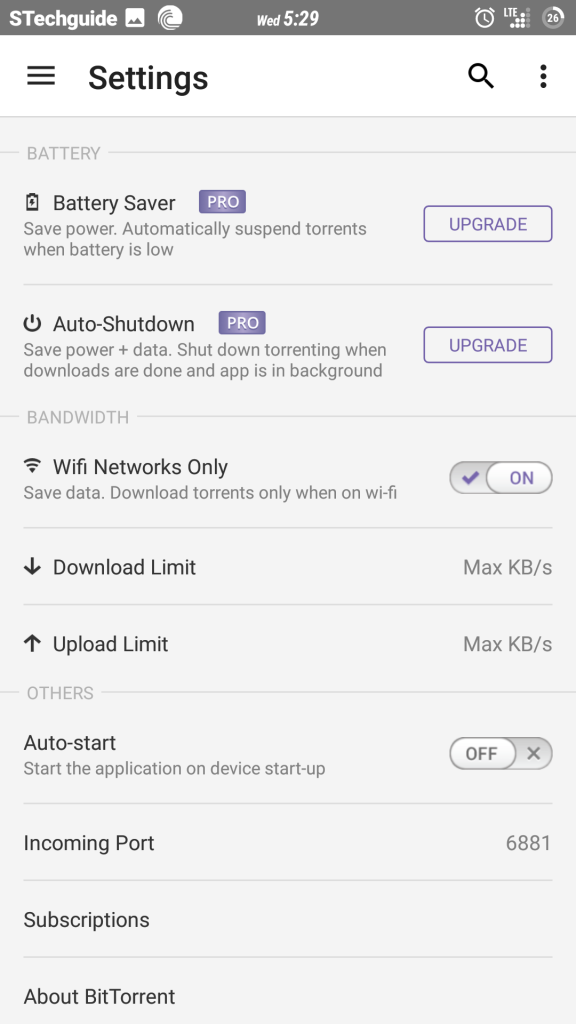This screenshot from a mobile phone displays a light gray background at the top, transitioning to a darker gray bar with white font text that reads "Tech Guide." Next to the text, there are two icons: a white gallery icon and a circular icon with a wave-like design. The time is displayed as "Wednesday 5:29" next to an alarm clock icon, a mobile signal icon with "LTE" above it, and a gray circle with a white "26" in the middle.

Beneath this, there is a large white rectangle on the left. Inside this rectangle, three vertical black bars are visible, followed by the word "Settings" in large black font. Adjacent to this are a magnifying glass icon and three vertical black dots, indicating more options.

The main content below features a gray page showcasing battery settings. At the top, the word "Battery" appears in light gray font, followed by "Battery Saver" in black font. Next to this is a small purple rectangle labeled "Pro" in white font. Below the text, there's an explanation: "Save power automatically suspends torrents when the battery is low." To the right, a rectangular button labeled "Upgrade" in purple font is present. Further down, the option "Auto Shutdown" is displayed.